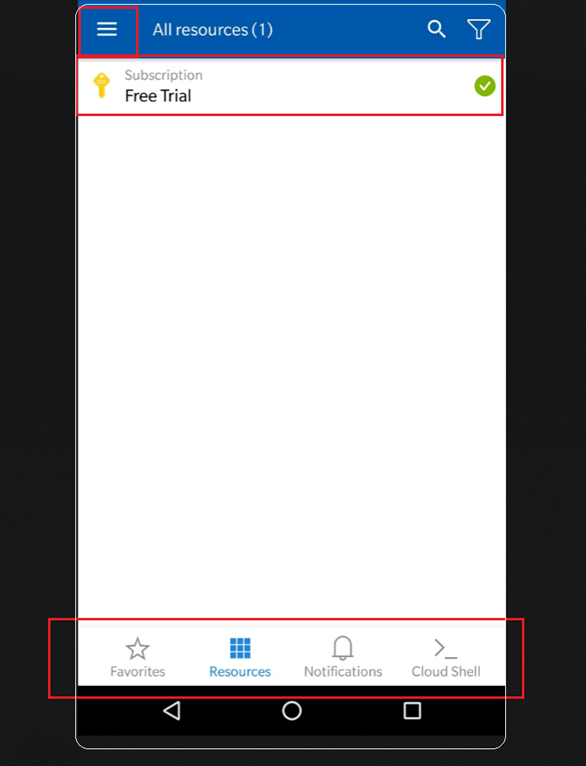The image appears to be the screen of a cell phone displaying an educational app interface. 

At the top of the screen, there is a horizontal red bar. On the left side of this bar, there are three white horizontal lines stacked vertically, representing a menu icon. To the right of this icon, the text "All Resources (1)" is displayed. Towards the far right of the red bar, there are icons for a magnifying glass, symbolizing a search function, and a funnel, indicating filter options. The red bar continues to form a rectangular frame around the three-line menu icon.

Beneath the red bar, the screen displays a white section containing the text "Subscription Free Trial." Adjacent to this text, there is a yellow key icon. Further to the right, a green circle with a white checkmark is shown, also enclosed within a red rectangular frame.

The majority of the remaining screen is white, featuring navigation options at the bottom labeled "Favorites," "Resources," "Notifications," and "Cloud Shell." These options are highlighted by a red rectangle. The "Resources" tab is colored blue, indicating that it is the active section of the app, while the other tabs are gray.

The sides of the image have black borders, and the bottom edge of the cell phone screen is also black, featuring navigational icons: a left-facing arrow, a circle, and a square. A white edge is present at both the top and bottom of the screen, helping to delineate sections of the interface for better visibility.

The detailed interface elements and navigational aids suggest that this app is being used for educational purposes, guiding users through resources and tools effectively.